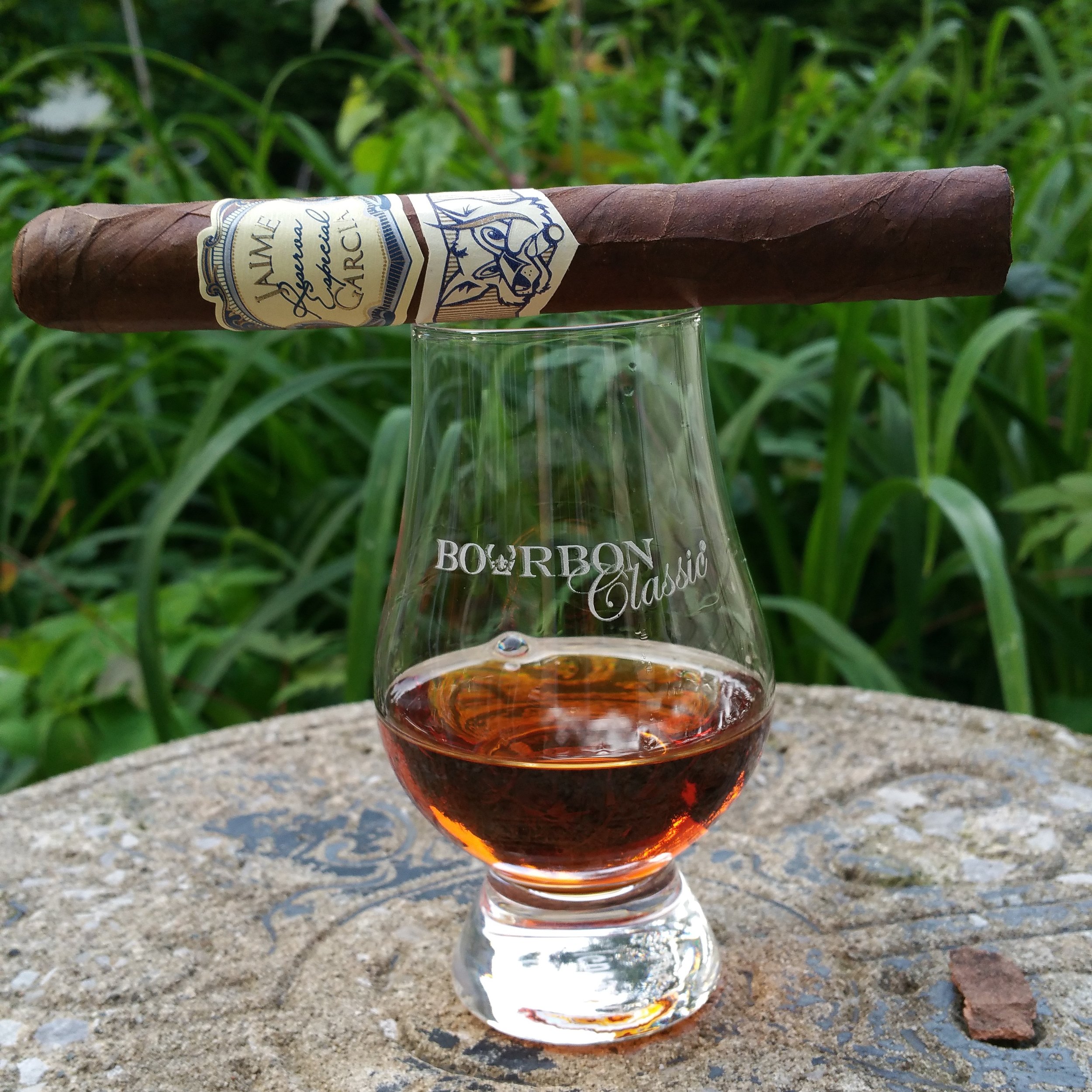In the image, a clear glass cup almost half-filled with a reddish-brown bourbon sits on a worn, circular platform that might be a log of wood or a stony table. The glass features the text "Bourbon Classic" engraved in white, with the word "Bourbon" in all capital letters and a decorative design on the "U." A large brown cigar, uncut, rests horizontally on top of the glass. The cigar’s label is white with intricate designs in light blue, darker blue, gray, and brown, featuring a fox or wolf smoking a cigar. The label also includes the text "Jaime Garcia Special Reserve." In the background, tall green grasses and leafy plants can be seen, enhancing the outdoor setting. There's a small piece of stone on the table, contributing to its weathered appearance with chipped paint or dirt revealing an older black surface beneath.